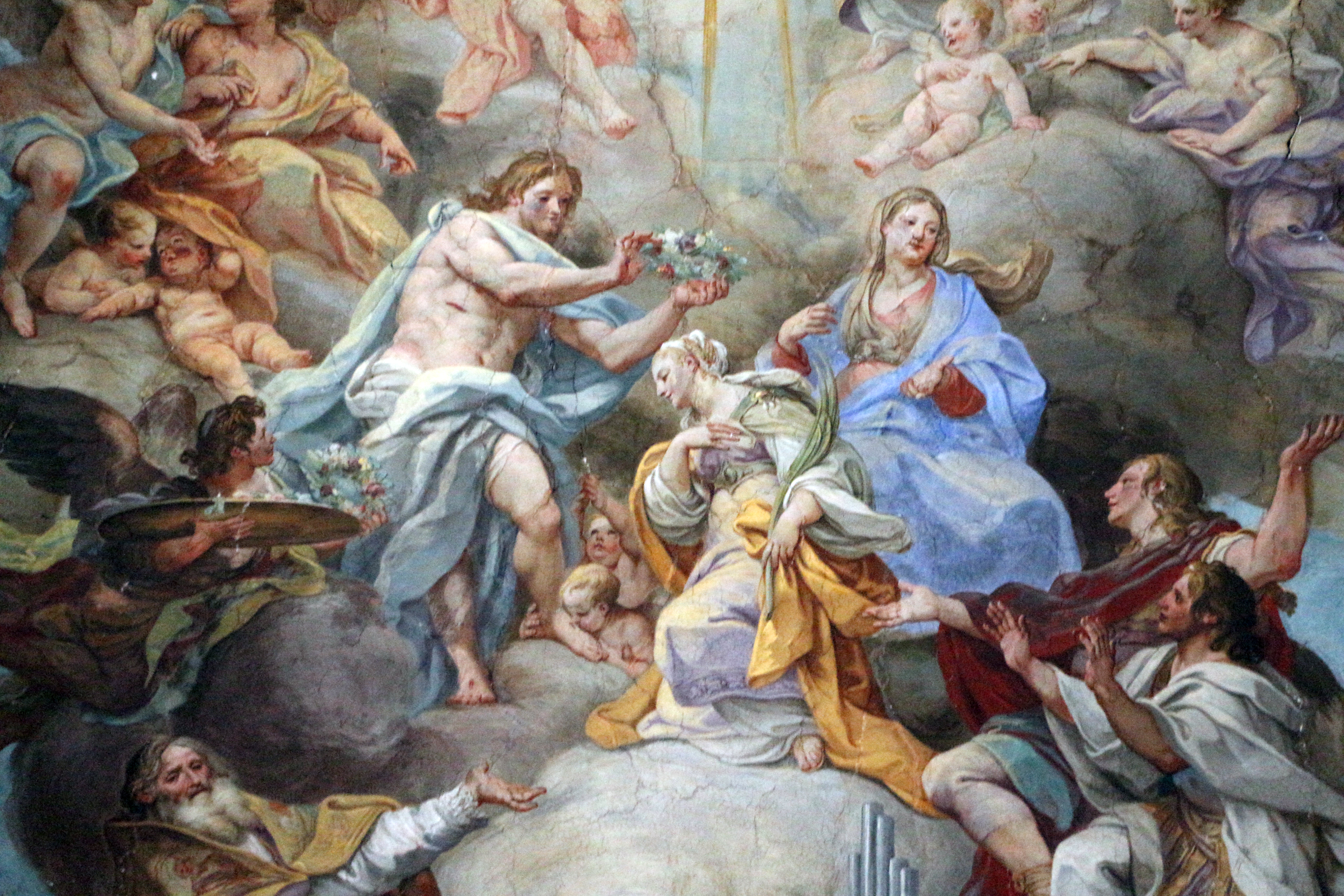The painting features a celestial scene where various figures are seated on white and tan-colored clouds, all directing their attention towards the center. Dominating this focal point, a man with flowing blue and white robes and an exposed chest is crowning a woman to his right with a wreath made of flowers and green leaves. This crowned woman, positioned centrally, is adorned in a white dress and a yellow shawl, her hair elegantly tied up with a white cloth. Adjacent to her, another woman clad in a blue robe over a red dress looks off into the distance; her hair is neatly wrapped in a tan cloth.

Floating above these figures are cherubs or angels, adding an ethereal quality to the scene. In the bottom left corner, an elderly man with a long white beard and outstretched arms stands, wearing garments with long white sleeves. Beside him, another individual gazes upwards, holding a board and some flowers. The overall composition of the painting suggests a historical or biblical theme, further emphasized by the presence of angelic beings and two striking gold lines descending through the backdrop. The use of clouds and heavenly ambiance reinforces the divine atmosphere of the artwork.